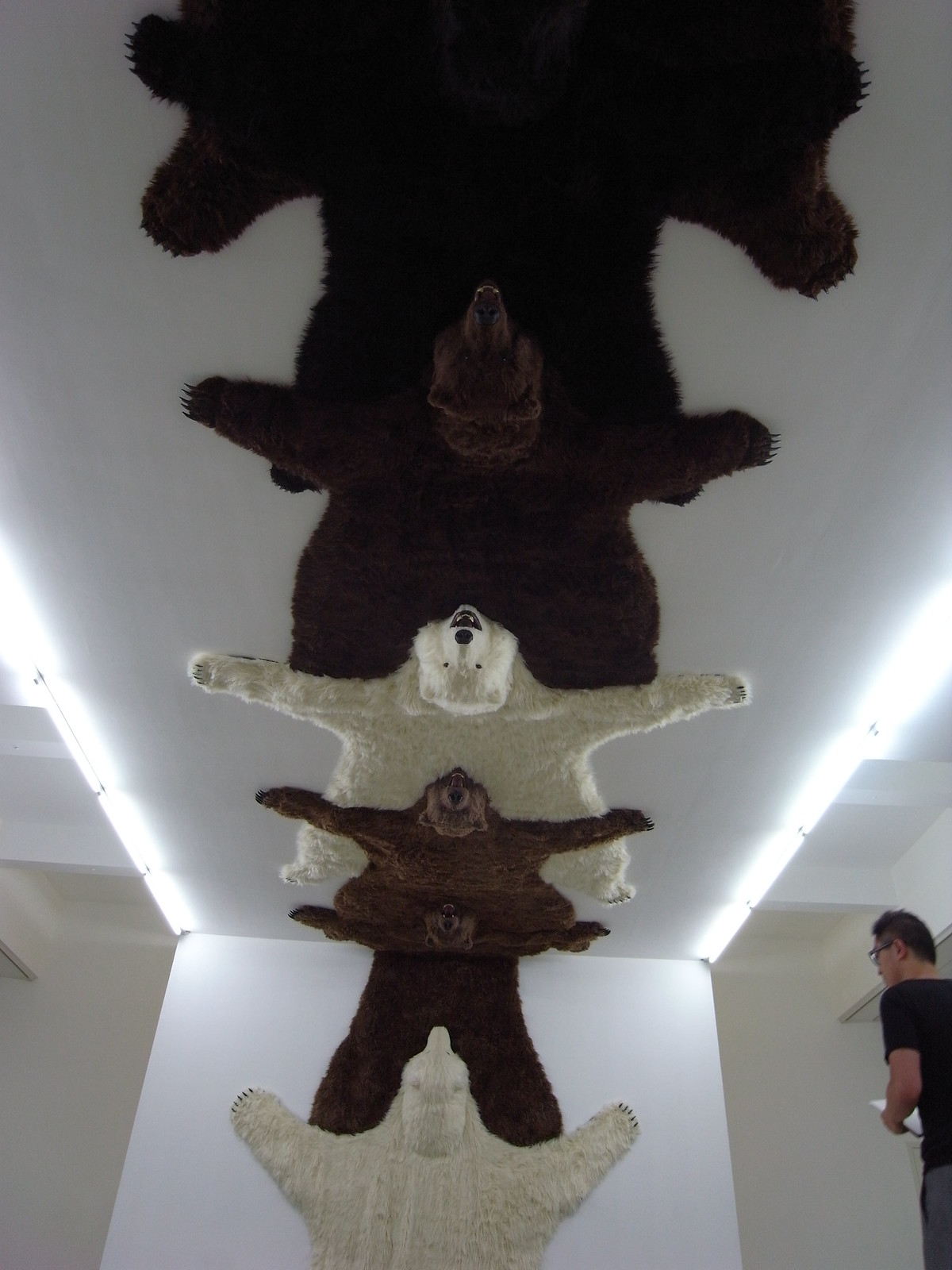In this intriguing photograph, the image captures a unique arrangement of several bear rugs, intricately draped from a wall extending up to the ceiling in a fascinating crotch-to-head pattern. The rugs, which appear to be made from carpet rather than real bear hides, feature both white (resembling polar bears) and varying shades of brown. From our upwards-looking perspective, we observe two rugs affixed to the wall, seamlessly connecting to five additional rugs that extend across the ceiling, forming a continuous line.

Distinctly, the heads and outstretched paws of these bear rugs are vividly visible, with particular clarity on five of them, creating an almost surreal decor. The photograph includes a man situated in the bottom right corner, dressed in a black t-shirt and glasses, seemingly engrossed in inspecting the array of bear rugs. He holds some paper in his hands and directs his attention particularly towards a white rug positioned at the base of the wall. The interplay of this unique display with the observer adds an element of curiosity and depth to the image.